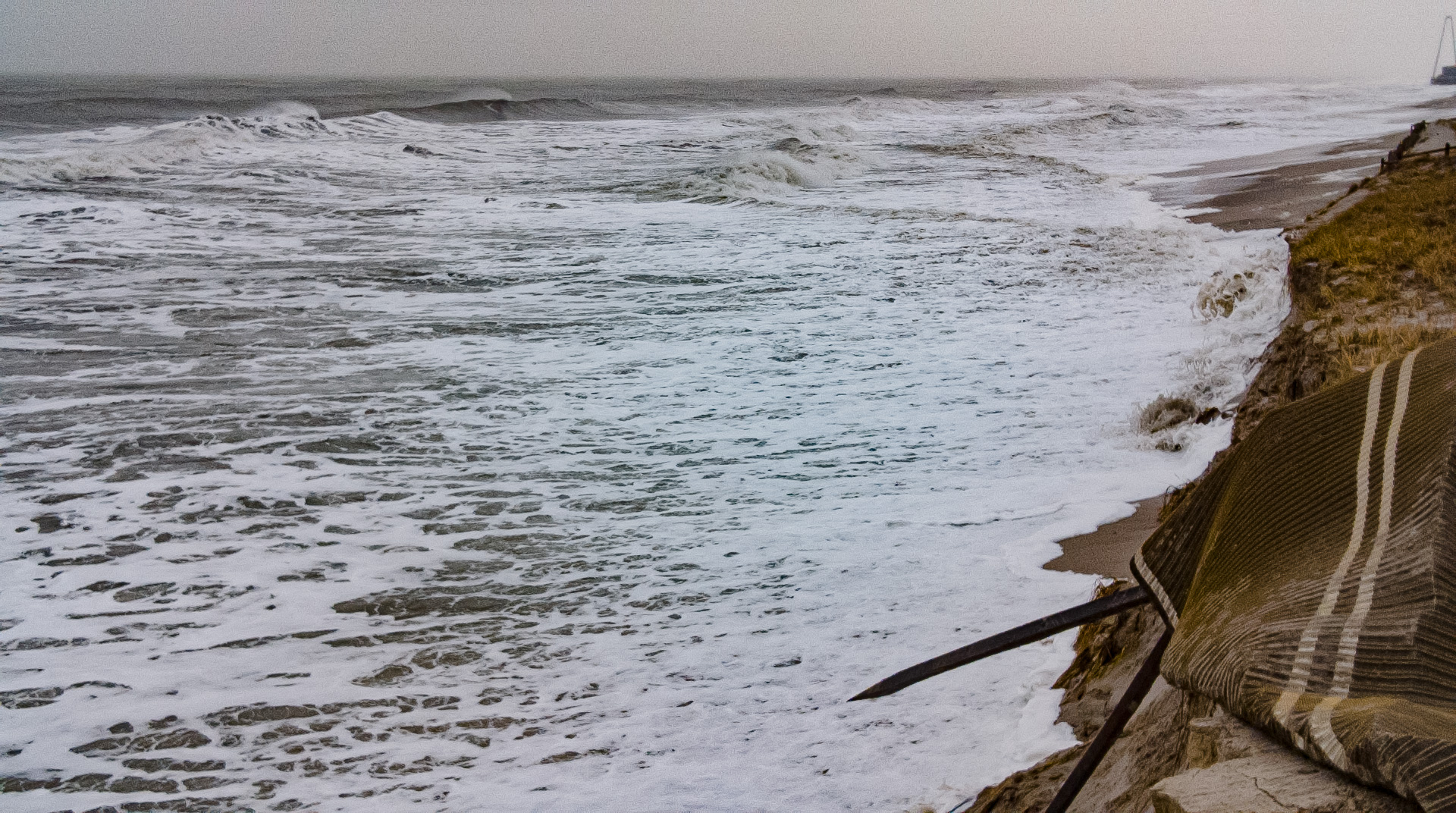The photograph captures a rough sea crashing against a beach during high tide, with tall, frothy waves dominating the scene and only a small section of the beach visible on the right. The waves are turbulent and filled with white foam, appearing to engulf most of the image. Above this tumultuous ocean scene is a narrow strip of horizon marked by a grey, overcast sky. Along the shoreline, patches of light green beach grass and some metal stakes hint at efforts to combat erosion. In the foreground, a brown striped sweater lies on the edge of what seems to be a cliff or elevated ground, suggesting the forces of the sea have ravaged the area. The entire scene is monochromatic, mainly subdued hues of grey, blue, and white, painting a picture of a cold, windy, and somewhat melancholic day.